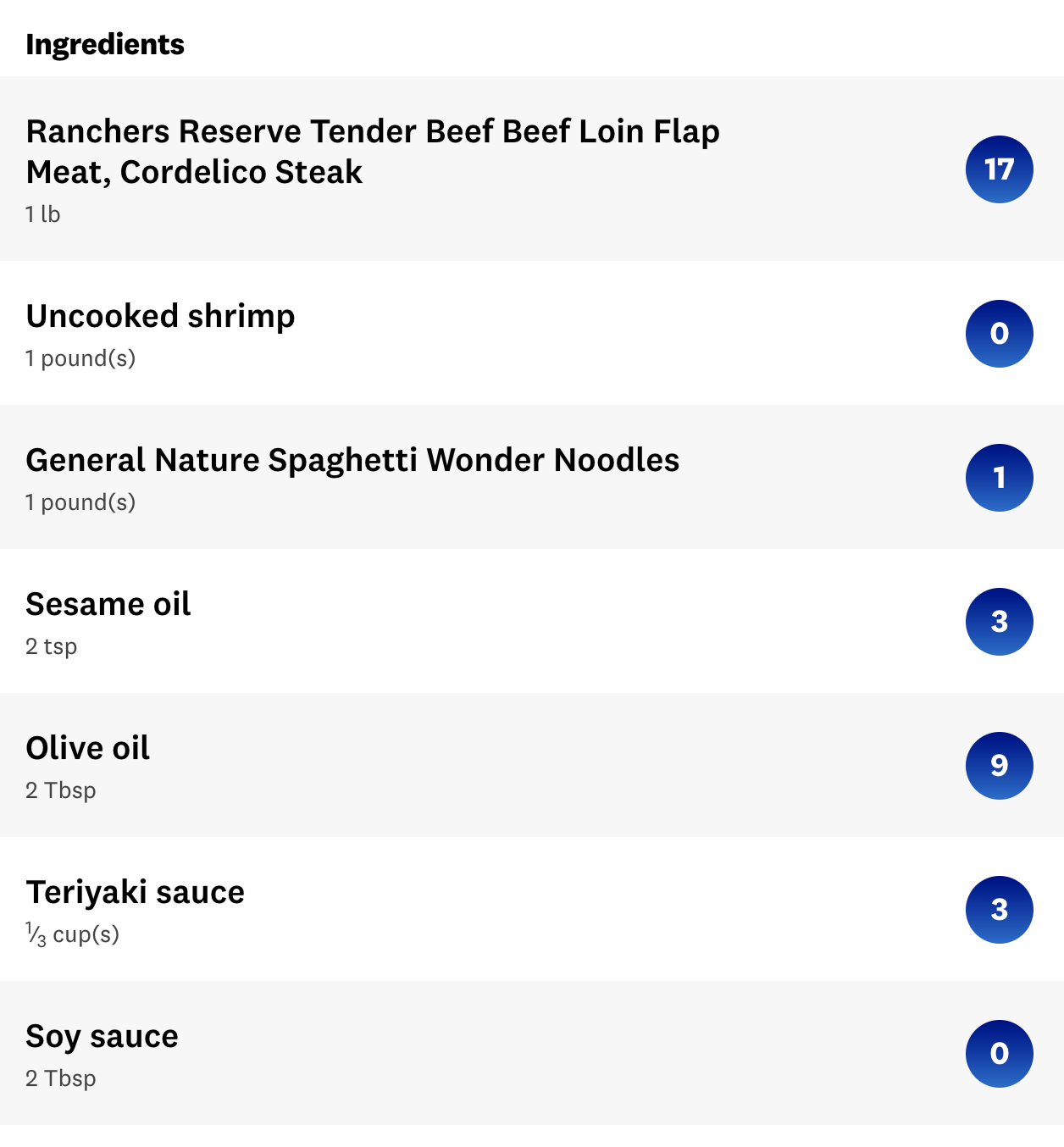This image features a detailed cooking list for a main course dish against a white background. At the top, "Ingredients" is prominently displayed in black text. Below, the ingredients are listed as follows:

- Rancher's Reserve Tender Beef Beef Loin Flap Meat Cordello Steak: 1 lb.
- Uncooked Shrimp: 1 lb.
- General Nature Spaghetti Wonder Noodles
- Sesame Oil: 2 teaspoons
- Olive Oil: 2 tablespoons
- Teriyaki Sauce: 1/3 cup
- Soy Sauce: 2 tablespoons

To the right of each ingredient, the necessary quantities are distinctly outlined within blue circles featuring a gradient from dark to light blue. The text within these circles is white, set in a serif font. The specific quantities are:

- Rancher's Reserve Tender Beef Beef Loin Flap Meat Cordello Steak: 17 lbs.
- Uncooked Shrimp: 0 lbs.
- General Nature Spaghetti Wonder Noodles: 1 lb.
- Sesame Oil: 3 tablespoons
- Olive Oil: 9 tablespoons
- Teriyaki Sauce: 3 tablespoons
- Soy Sauce: 0 tablespoons